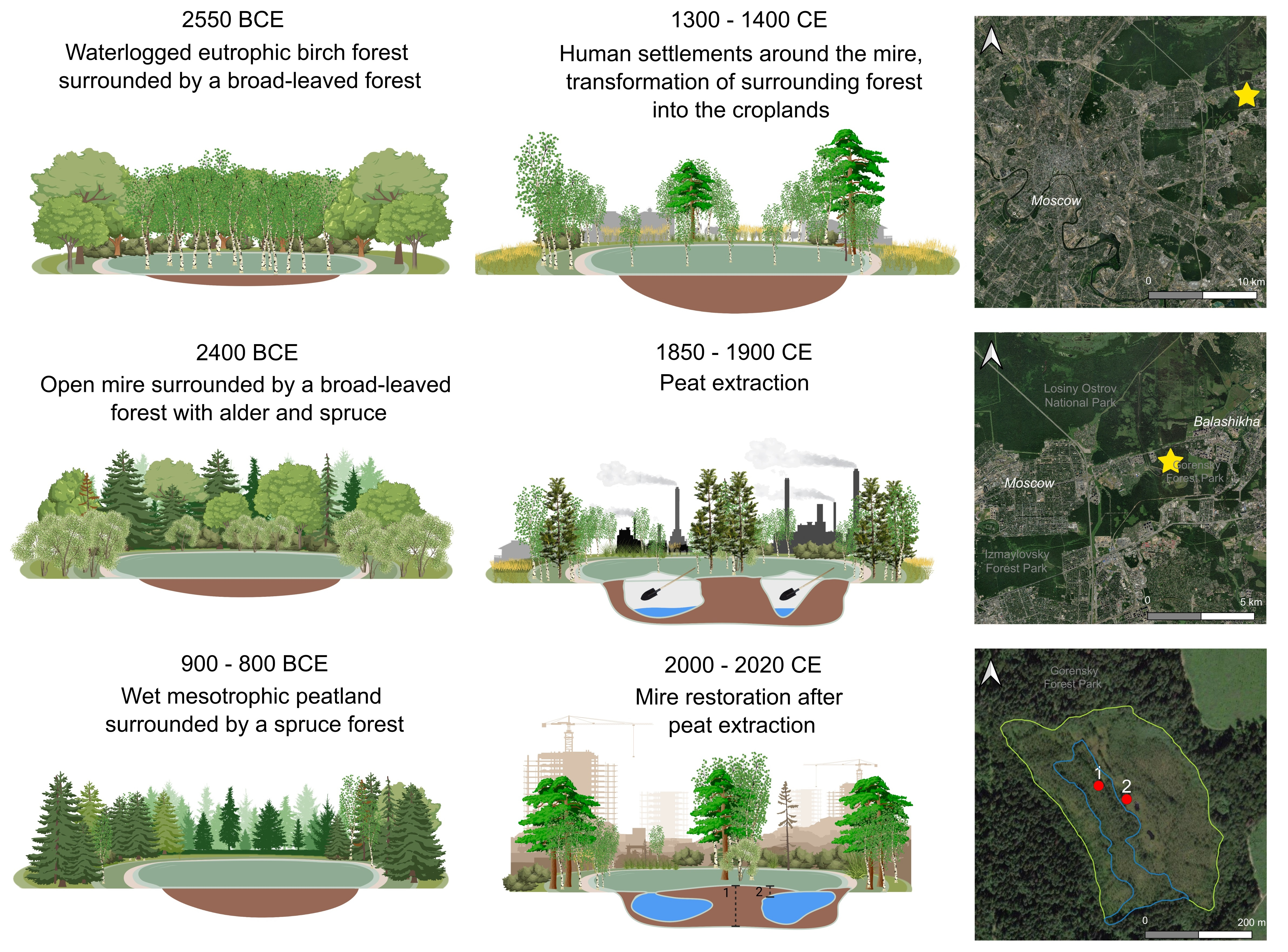The teaching poster features a timeline illustrated with nine images depicting the transformation of a forest ecosystem from 2550 BCE to the present day, including different stages of marshland and human influence. On the left side, six sequential images detail significant periods: starting with a waterlogged eutrophic birch forest surrounded by broad-leaved trees, moving through stages of human settlement and agricultural transformation around the mire, the dominance of alder and spruce in open mires, and then to a wet mesotrophic peatland surrounded by spruce forest (900-800 BCE). The timeline covers the major historical changes in land use, including peat extraction in the 19th century, and concludes with the mire restoration phase in recent times (2000-220 CE). Highlighted are the transitions from dense, leafy forests and marshlands to croplands and back to restored mires, punctuated by visible human activity such as houses and infrastructure. On the right side, three satellite images, possibly of Moscow, provide contemporary geographical context and contrast to the historical progression on the left. The poster's detailed evolution underscores the dynamic interaction between natural landscapes and human development over millennia.